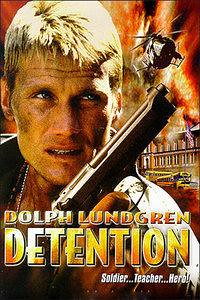This image features a striking advertisement for a movie. Dominating the left side is a man with spiky blonde hair and light-colored eyes, his face marked with smudges of yellow and red, conveying a weathered, gritty appearance. He holds a handgun diagonally across the center of the image, pointing it to the upper right while looking in the same direction. He wears a serious and alert expression, and a chain hangs around his neck, adding to the rugged, action-hero aesthetic.

In bold, gold letters at the bottom, the text reads "Dolph Lundgren," followed by "Detention" in larger text beneath, emphasizing the movie title. Lined up on the lower right in smaller white letters, the words "Soldier," "Teacher," and "Hero" describe Lundgren's character.

The right side of the background adds to the action-packed scene with a fiery explosion behind a helicopter at the top. Below, there is a large, two-story building and a long structure accompanied by two school buses positioned at the bottom, hinting at a dramatic and chaotic scenario.